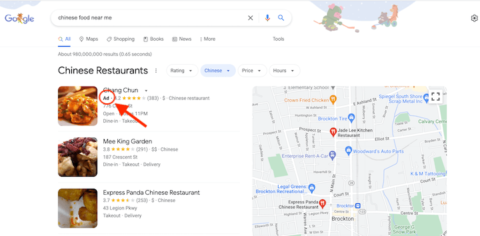This screenshot captures a Google search results page with a prominent, white background. The header features a whimsical cartoon illustration: an undulating white hill set against a light blue sky. On the hill, two cartoonish creatures are engaged in a sport resembling hockey, positioned near the bottom right of the image. To the left of this illustration is the iconic Google logo in blue.

To the right of the logo is the search bar, designed as a white rectangle with rounded ends and a light gray shadow, where the search query "Chinese food near me" is typed in black text. Adjacent to the search bar on the right side, there is a gray "X" icon, followed by a microphone with a red base and blue top, and a blue magnifying glass icon.

Below the search bar, the page displays several tabs, with a highlighted category for "Chinese restaurants." The search results showcase three listings, each with an image on the left and corresponding details on the right. The top listing is for a restaurant named "Changchun," which is distinctly marked by a bolded word with an "Ad" label. This label is emphasized further by a red circle and an arrow pointing from the bottom right, partially obstructing some of the restaurant's details.

To the right of these listings is a map, showing a network of white streets. The map is populated with pins in various colors – blue, red, gray, and orange – each accompanied by matching text labels, indicating different locations related to the search query.